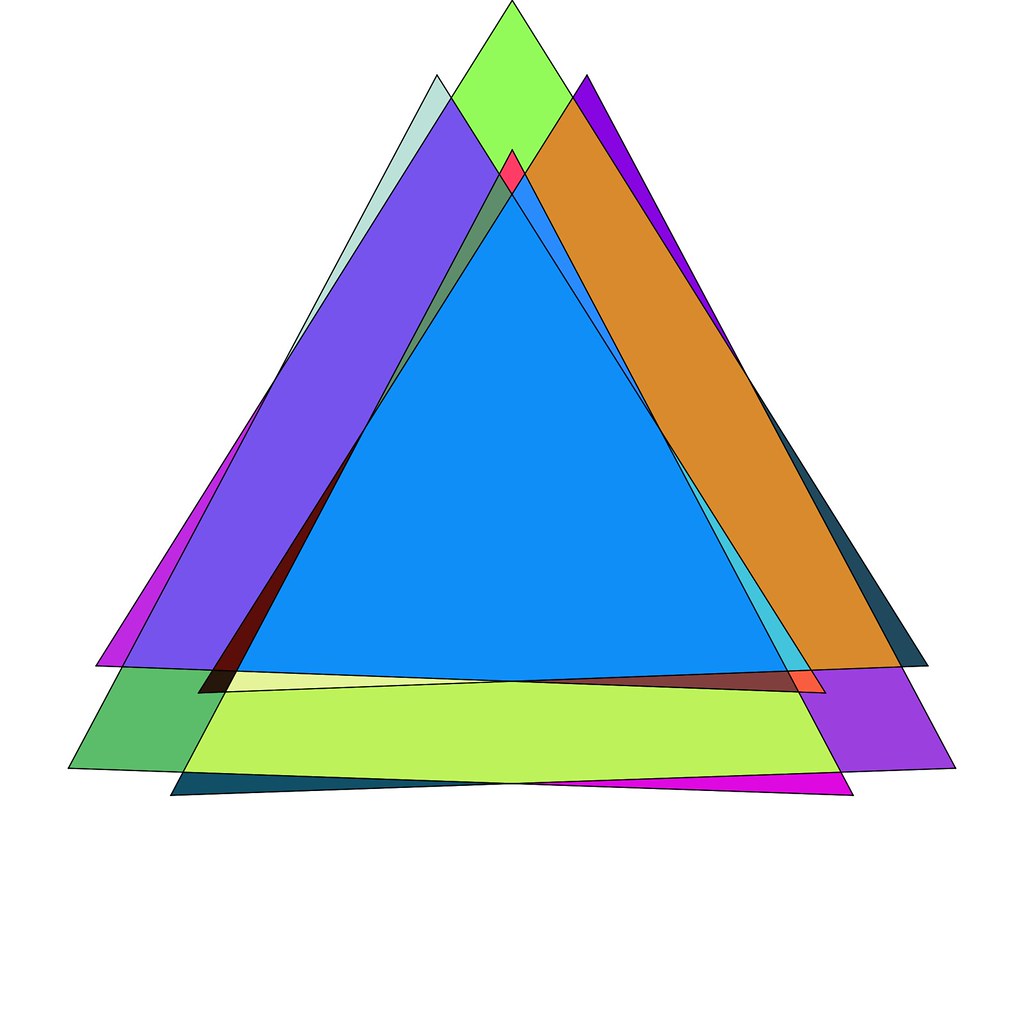The image presents an abstract composition of numerous colored triangles overlapping against a white background. The arrangement forms a shape reminiscent of a mountain peak. At the summit, there's a light green triangle, beneath which is a small diamond-like shape, resembling a volcanic eruption. Below this, two blue triangles, and bits of brown and cream triangles are visible. Further down, an olive green triangle overlies dark blue and pink triangles. On the left side, a prominent purple triangle is accompanied by a lighter purple one and a dark green triangle at the bottom left. A small grey sliver is seen above the dark purple triangle. Towards the right, a turquoise triangle and an orange triangle stand out. The entire layout suggests around eight to ten triangles in various sizes and colors, including shades of purple, violet, dark teal, light and dark greens, blues, pink, brown, cream, grey, turquoise, and orange. Each triangle has a distinct, dark black border, and their overlapping creates multiple jagged edges and overlapping colors, making the individual shapes partially visible while forming an intricate and dynamic visual pattern. The triangles' intersections and the clear white backdrop emphasize their colorful array, creating a striking visual focus on the varying sizes and hues of the triangles.